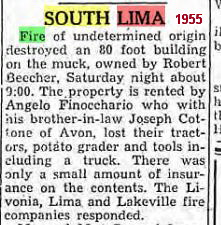This image features a small, slightly blurry newspaper clipping with a focus on a news article titled "South Lima, 1955." The title "South" is highlighted with either a white or yellow background, and "Lima" is emphasized with a red or dark orange/light pink background. The year "1955" is distinctly printed in red font. The article begins with the word "Fire," highlighted in green, and goes on to detail an incident where an 80-foot building on the muck, owned by Robert Beecher, was destroyed by a fire of undetermined origin at around 9 p.m. on a Saturday night. The building, rented by Angelo Finocchario, who with his brother-in-law Joseph Cottone of Avon, lost tractors, a potato grader, tools, and a truck in the fire; there was minimal insurance covering the contents. The Livonia, Lima, and Lakeville Fire Companies responded to the emergency. The article is part of a larger clipping, but the remaining text is cut off and unreadable.